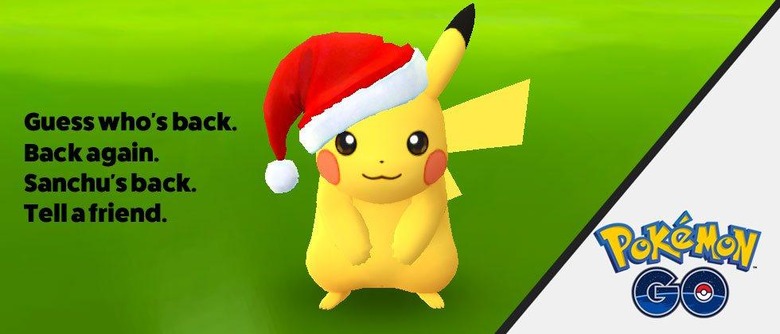This charming image of Pikachu from Pokémon features a festive design. The background is divided into two sections; three-quarters of it is lime green with a darker green base, while the remaining quarter is light gray. At the bottom right of the light gray section, the words "Pokémon GO" are prominently displayed, with "Pokémon" in yellow and "GO" in navy blue, including white and maroon accents inside the 'O'. 

Occupying the lime green portion of the image is Pikachu, adorably dressed in a Santa hat that sits diagonally on his head, causing one ear—tipped in black—to stick out. Pikachu's festive look is complemented by his signature red circular cheeks and inquisitive gaze directed straight at the viewer. Beside Pikachu, a playful message is written in bold black letters: "Guess who's back, back again, Sanchu's back, tell a friend!" This cheerful holiday-themed image captures the spirited essence of Pikachu from the beloved Pokémon series.